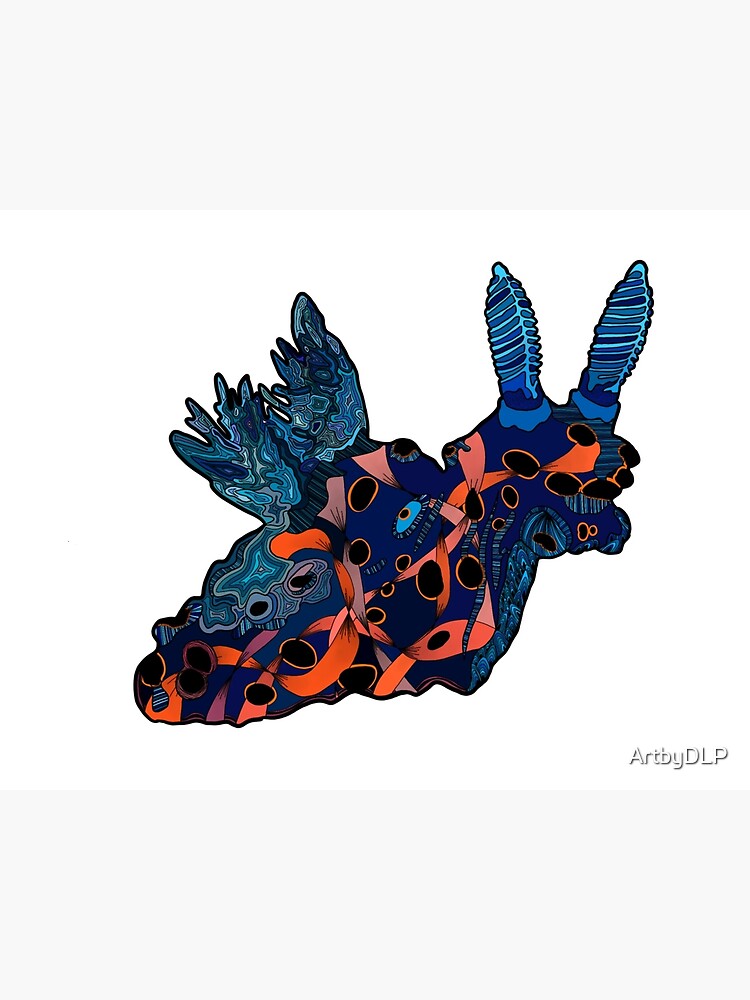The image is a tall, digitally illustrated graphic design featuring light gray rectangles functioning as borders at the top and bottom, framing a primarily white background center. Dominating the composition is an abstract creature-like form moving to the right. The creature, outlined in black, resembles a snail with additional features that evoke bunny ears or moth antennas. Its body is predominantly navy blue, adorned with intricate patterns and textures. Short, bluish wings, seemingly feathered with central ribs and lines radiating outward, extend from its back. Orange-red ribbons weave through the form, adding dynamic movement. Black, oval shapes outlined in orange punctuate its blue expanse. The bottom right corner bears a white text signature, "Art by DLP," with a black drop shadow, adding to the piece's mystique.